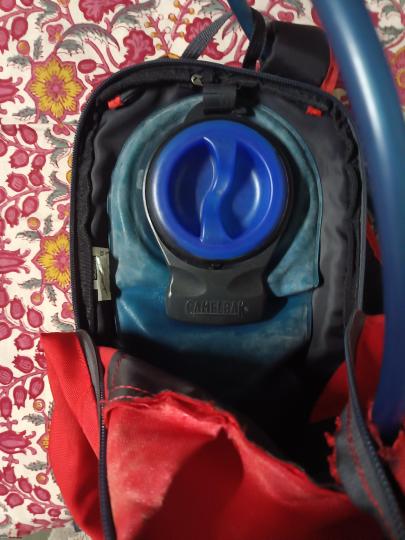The image is a color photograph, oriented in portrait, capturing a detailed view of a CamelBak hydration backpack. The primary focus is on the bag, which is positioned near the top half of the image. The bag features a black nylon rim and a blue inner lining. At the center, there's a black plastic disc adorned with a blue screw-on lid for filling the water reservoir. This lid is equipped with finger grips on each side to facilitate opening. The top portion of the bag also includes several straps for securing it, along with a distinctive black tab for flipping open the lid.

The exterior of the bag showcases a vibrant color scheme: the top is black, while the bottom half is red, folded slightly downwards. A prominent blue tube, used for drinking, runs from the water reservoir up the right side of the bag, exiting the top right corner. This tube features a nozzle at the end for easy drinking while on the move.

The bag is laying on a surface that appears to be covered with a floral-patterned tablecloth or wallpaper, which has a white background adorned with yellow flowers and red vines. The overall style of the photograph is representational realism, providing a clear and precise depiction of the CamelBak hydration backpack in its environment.